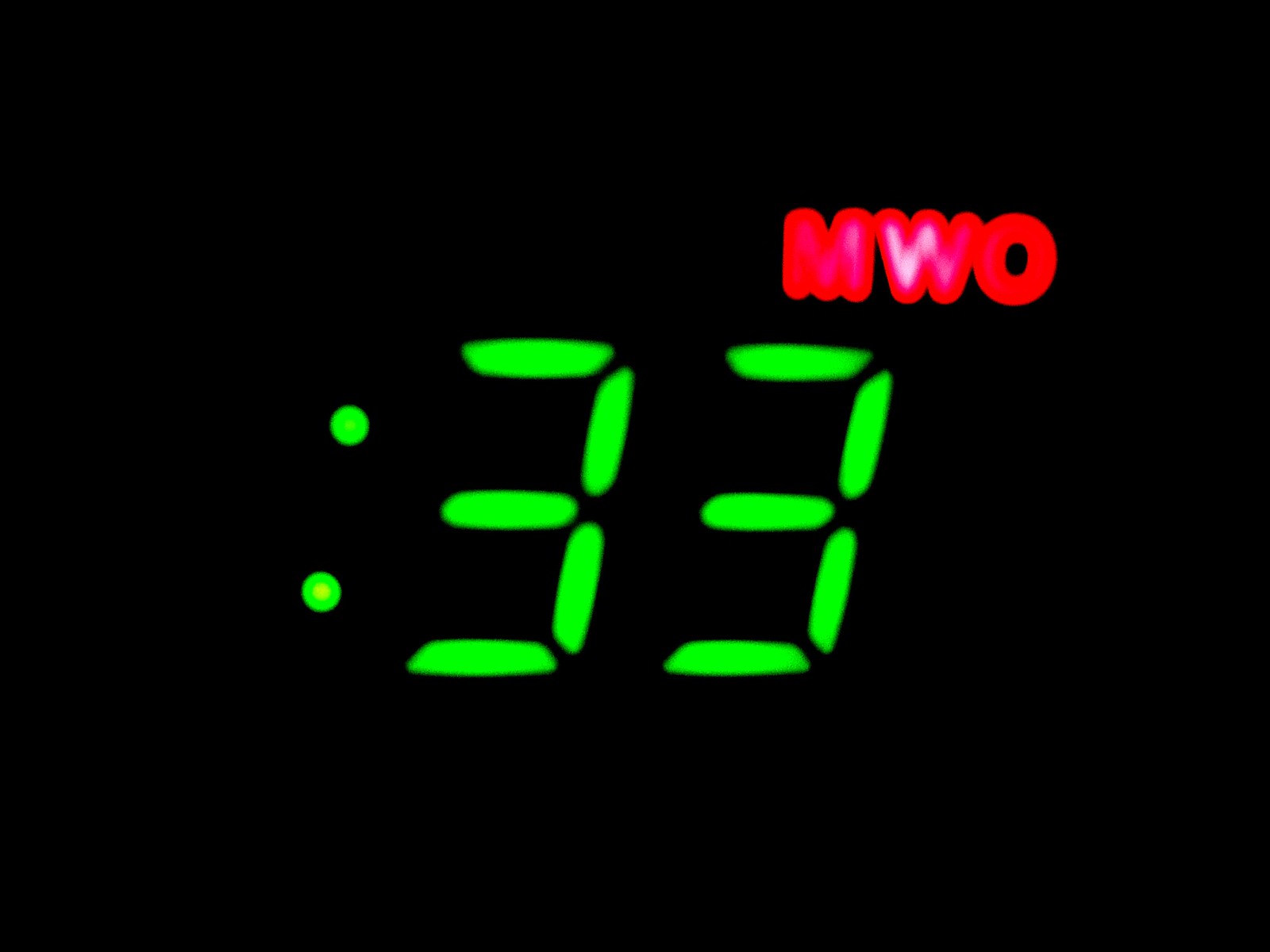This image displays a digital readout against a completely black background. Central to the image are two green, broken numbers "33," resembling the segmented digits of an LED clock. Positioned to the upper right of the numbers are the letters "MW," rendered in red, with the "W" having a subtle white reflection in its center, suggesting an external light source aside from the inherent illumination of the characters themselves. The two dots indicating time between the numbers "33" further suggest the possibility that the image is denoting 33 seconds. No additional time indicators are present to the left of the dots, leaving the exact nature of the time measurement ambiguous. The stark contrast between the vivid green and red characters and the black background creates a striking visual.